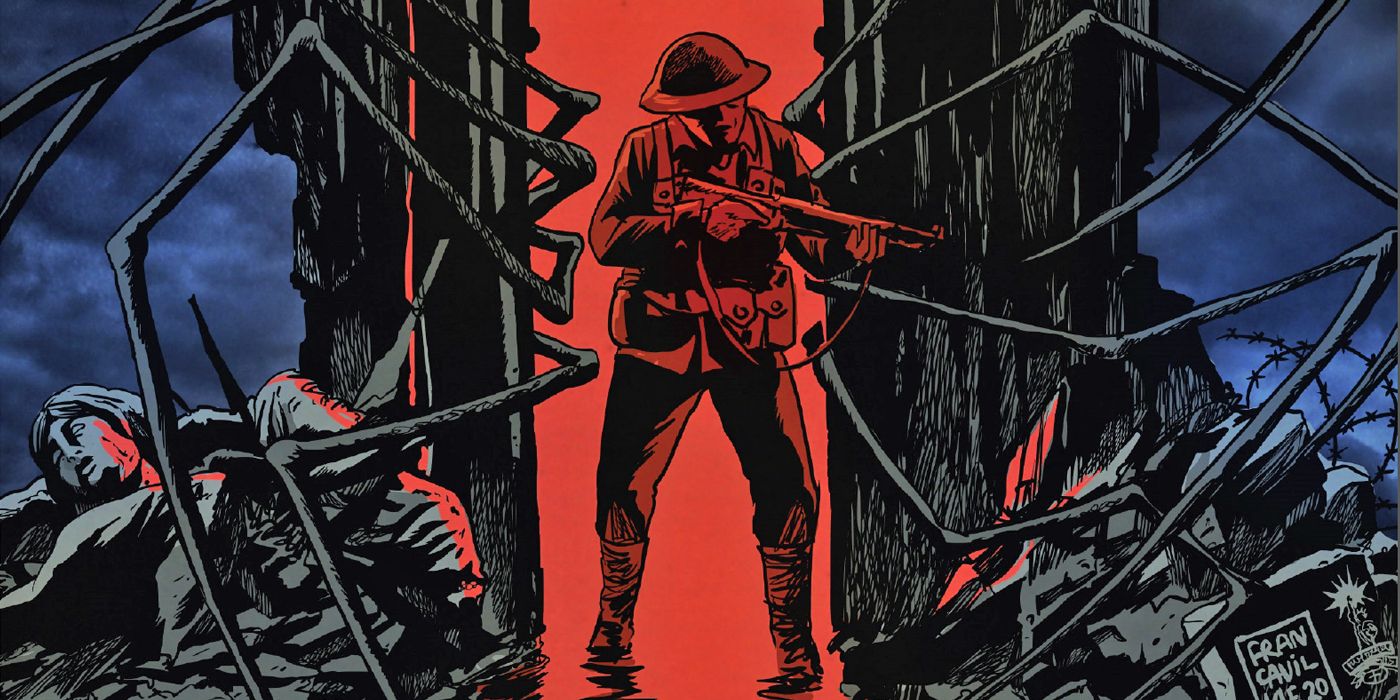The illustration features a stark, limited color palette dominated by thick lines and heavy shadows. In the center stands a soldier, fully illuminated in red against a black structure, suggesting a night scene under a dark blue sky with gray clouds. The soldier, whose uniform hints at East Asian origins, wears a round-topped helmet with a short brim. He holds a rifle pointed toward an unseen target on the lower right.

Positioned in a doorway, the soldier is flanked by spider-like legs emerging from the doorway, extending towards the edges of the image, creating an eerie atmosphere. This central figure is surrounded by contrasting details: on the left, a dead woman with long hair lies atop a pile of debris, rendered in gray and black with red splotches likely cast by the soldier's illumination. On the right, another pile of indeterminate debris is similarly shaded in gray and black.

Despite the macabre scene, the background showcases a dark, almost nightmarish blue sky, punctuated by ominous gray clouds. In the bottom right corner, the artist's signature, handwritten in pale gray, reads "Fran Caffin," adding a personal touch to this haunting composition.